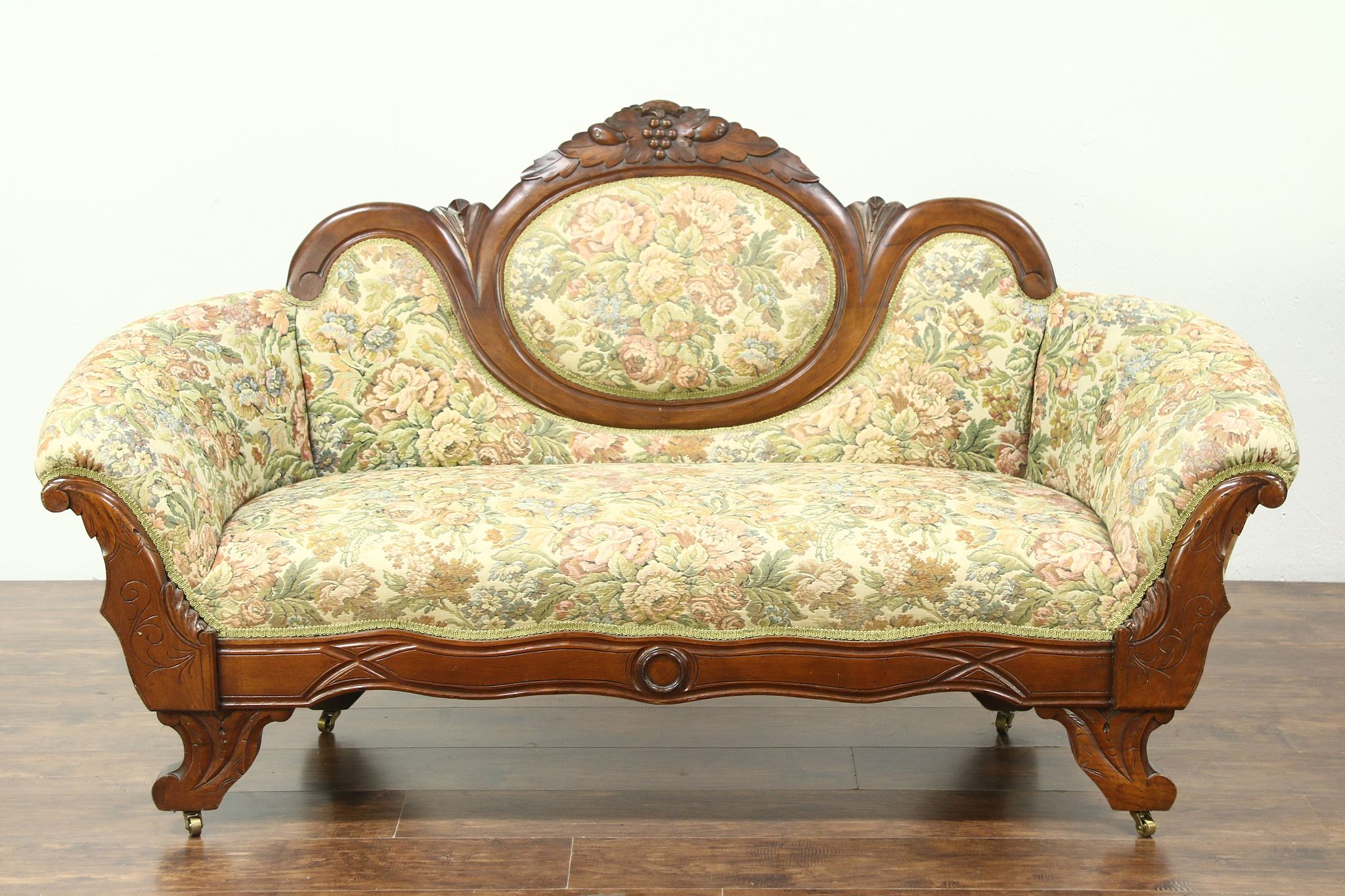In this professional photograph, a vintage-style loveseat is showcased against a pure white background, emphasizing its elegant design. The floor beneath it is a dark, handcrafted wooden surface, adding to the overall antique aesthetic. The loveseat itself features a beautifully carved dark wooden frame, adorned with leaf and grapevine motifs at the top, contributing to its ornate appearance. The backrest includes an oval wooden frame with a matching cushion inside, covered in a green and yellow floral-patterned fabric, with pink and orange flowers that vividly contrast against the darker wood. The loveseat, which appears capable of seating up to three people, is also designed with wheels on each leg, making it easily movable. This piece, possibly from the early 1900s, combines functionality with traditional charm, embodying a timeless elegance.